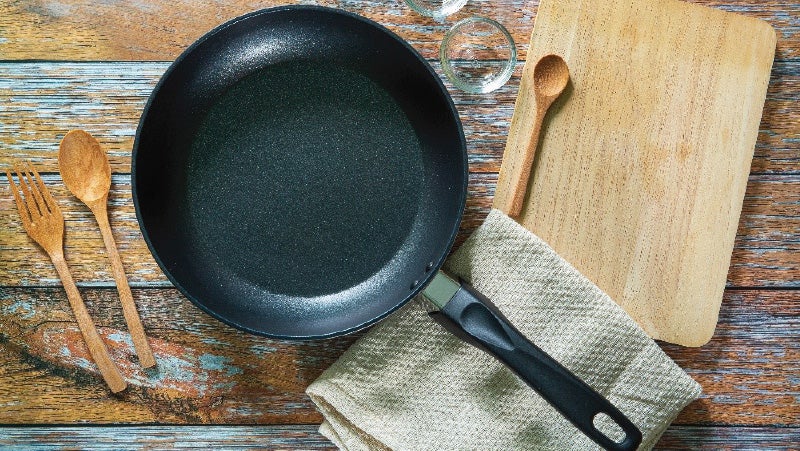This photograph captures a rustic kitchen setup centered on a distressed wooden table with hints of brown, blue, and gray tones. Anchoring the scene is a pristine, black non-stick Teflon frying pan with a black handle, positioned in the middle. Beneath this handle lies a neatly folded beige or cream dish towel. To the right of the pan, a brown wooden cutting board hosts a smaller wooden spoon, adjacent to which sits an empty clear glass or small glass bowl. On the left side of the pan, a larger wooden spoon and a wooden fork can be found, laid out and ready for use. Just above the cutting board, barely peeking into the frame, is the edge of another small glass container, its contents indeterminable. The arrangement suggests a moment of culinary preparation amid a beautifully textured wooden backdrop.